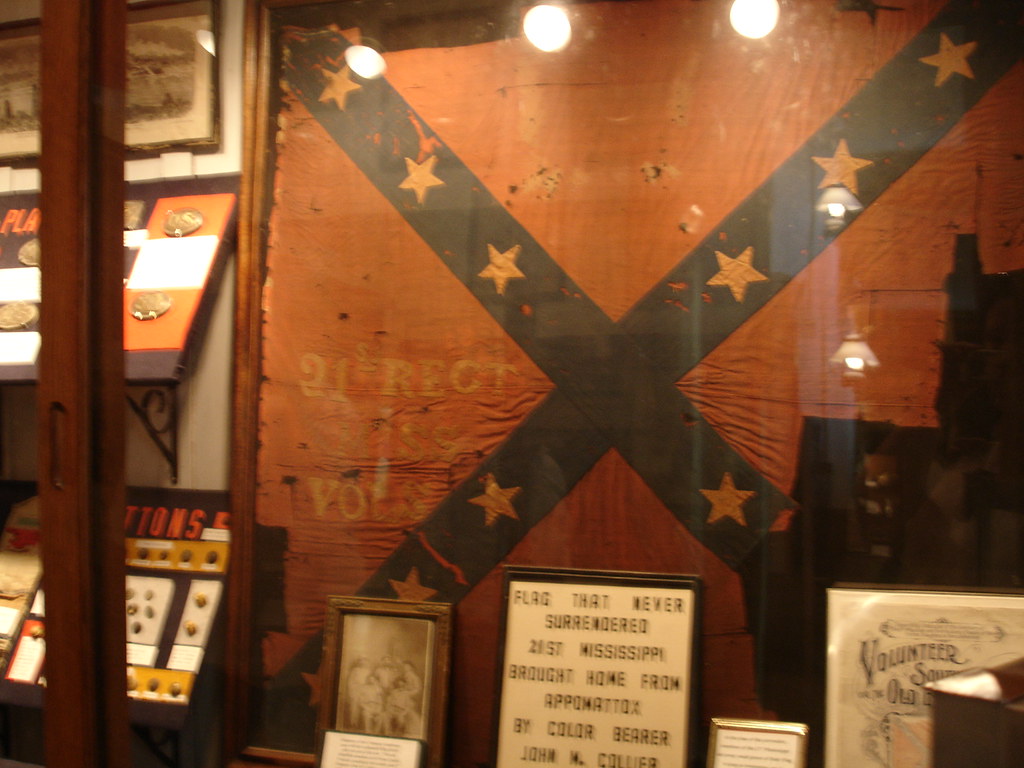The image depicts a detailed Confederate display, likely within an old museum, focusing on a prominent Confederate flag. The flag, characterized by an orange background with a blue X adorned with stars, is painted on an aged wooden surface. Below this flag is a significant framed image captioned, "Flag that never surrendered, 21st Mississippi, brought home from Adipatamax by color bearer John M. Collier," emphasizing the historical context. Surrounding the central flag and framed caption are various Confederate memorabilia, including black-and-white photographs and medals, meticulously arranged on shelves. These shelves appear to contain awards and plaques, possibly from wartime achievements. The entire display is encased in a protective glass unit, with the person's reflection faintly visible in the glass, indicating it is being observed from behind this barrier. The juxtaposition of these detailed artifacts adds to the authenticity and historical richness of the exhibit.